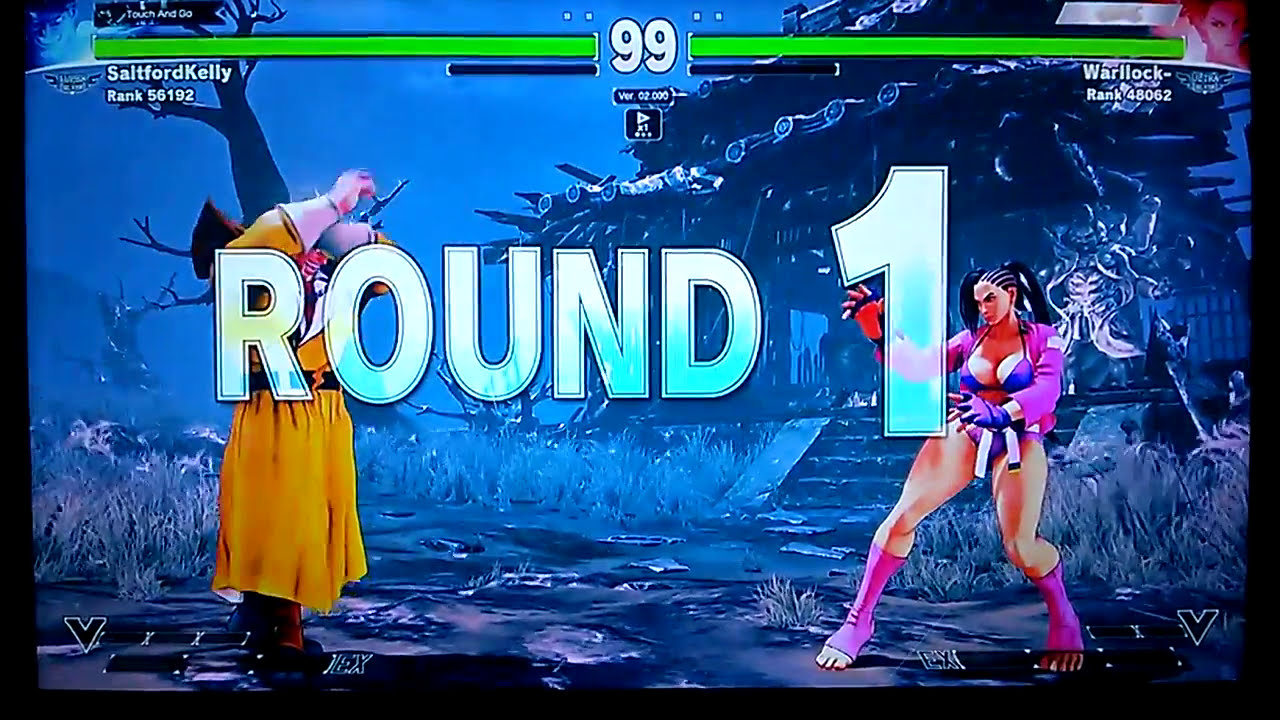This screenshot from a fighting video game captures the intensity of an imminent battle in "Round One," as displayed prominently in large white lettering across the screen. The background is steeped in ominous blue and gray tones, featuring a decrepit, rickety wooden building on the right and a dead, barren tree on the left, contributing to the eerie atmosphere. The left side foreground showcases a male character in a yellow robe with his arms raised in a blocking gesture, his face obscured from view. On the right, a young woman stands in a fighting stance with cornrows and a ponytail, clad in a purple bikini, pink jacket, and matching pink leg warmers. At the top of the screen, two green rectangles flank the number 99 in white, indicating the timer. Below the left green rectangle, the name "Saltford Kelly" along with the rank 56192 is displayed, while under the right rectangle, the name "Warlock" with the rank 48062 can be seen. This scene sets the stage for the first round of a thrilling combat encounter in the game.